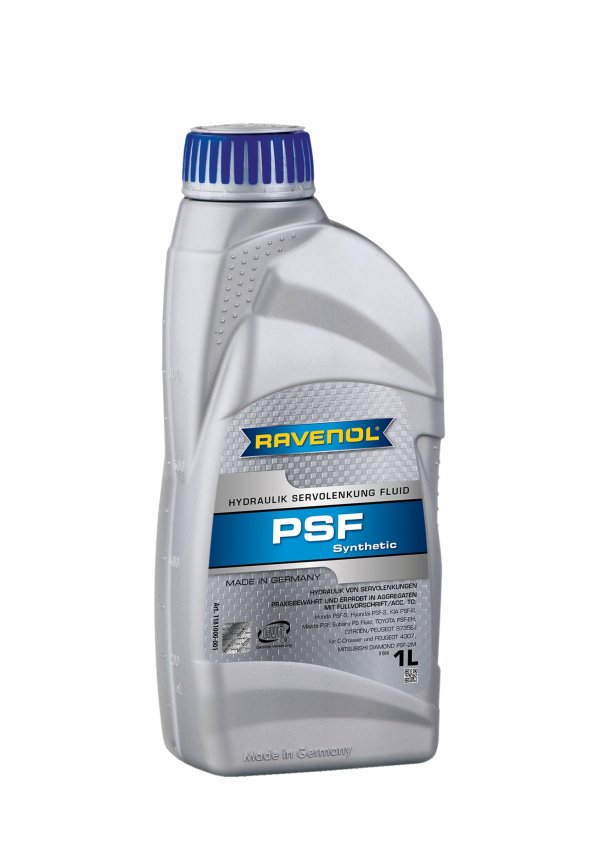This image displays a detailed view of a gray Ravenol hydraulic servo fluid container, specifically the PSF Synthetic type. The bottle is ergonomically designed for easy handling, with a predominantly silver body and a blue twist cap. The central label features the brand name "Ravenol" in prominent yellow text set against a blue banner. Below this, "Hydraulic Servo/Fluid" and "PSF Synthetic" are clearly marked. Additional markings indicate that the product is a 1-liter container and is made in Germany. Notably, there are raised measurement lines along the side of the bottle, aiding in determining the remaining fluid. The background of the image is plain white, emphasizing the bottle's sleek and functional design.